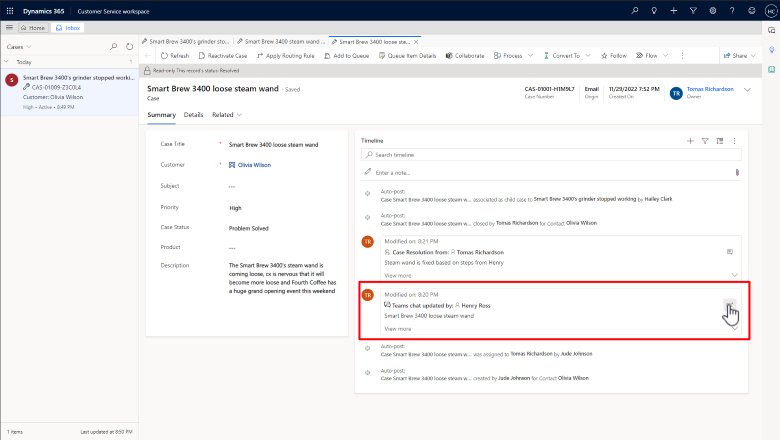A screenshot of a customer support portal addressing a reported issue with the SmartBrew 3400 coffee maker. The portal prominently displays the case number at the top for reference. The main title reads, "SmartBrew 3400 Loose Steam Wand," indicating the nature of the problem. Below the title, a detailed customer comment expresses concern: "The SmartBrew 3400 steam wand is coming loose. I'm nervous that it will become more loose." The screenshot captures the essence of a customer seeking assistance for a product defect through the portal interface.